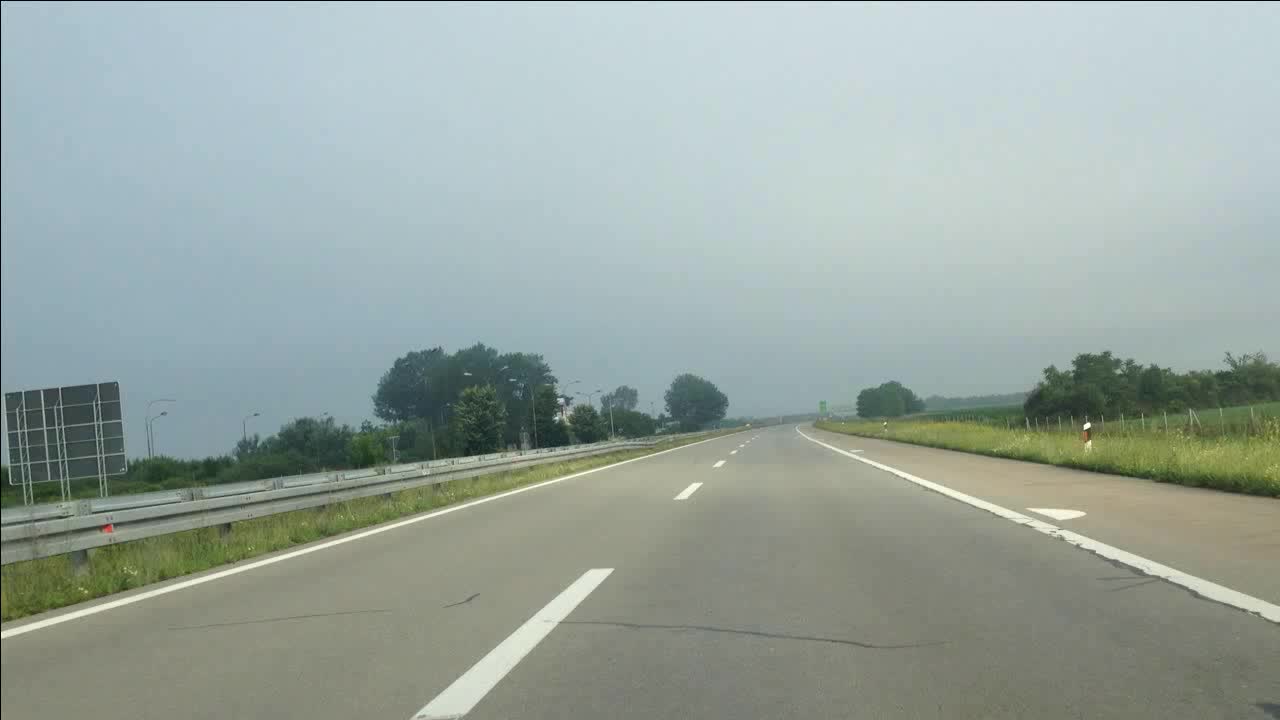The image depicts a serene highway scene enveloped by nature. On either side of the asphalt road, dense foliage and clusters of trees create a leafy green corridor. To the left, the back of a highway sign is visible, supported by sturdy metal bars. A broken white line demarcates the center of the road, interrupted by a discernable crack running across the asphalt. The road shoulder is clearly separated by a solid white line. Majestic, towering trees rise in the background, forming a thick, verdant canopy that frames the scene. The image captures the tranquil beauty of a roadway seamlessly integrated into its lush, natural surroundings.